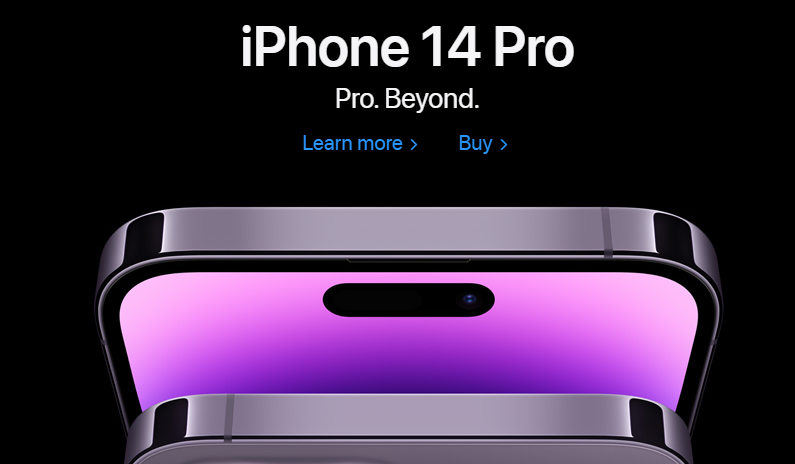The image is a screenshot of an advertisement for the iPhone 14 Pro, set against a completely black background in landscape orientation. At the top center, in bold white text, it reads "iPhone 14 Pro." Directly beneath that, in smaller, bold white text, it says "Pro. Beyond." 

Moving further down, there are two blue hyperlinks: "Learn more →" and "Buy →." 

At the bottom of the image, there are two prominent visuals of the iPhone 14 Pro. The first image, placed almost from the left of center to the right of center, shows a sleek outline of the iPhone with a silver edge. The phone has two distinct black areas on its sides, with only a partial view of its screen at the bottom. Behind this, the second, larger image seems to depict the iPhone 14 Pro as well, but this model has a vibrant violet screen and a noticeable black bar at the top center.

The visual setup suggests a transition from the smaller phone to the larger, more advanced version, implying that the new iPhone 14 Pro offers superior features and a more enhanced experience, signaling an upgrade necessity from previous models.